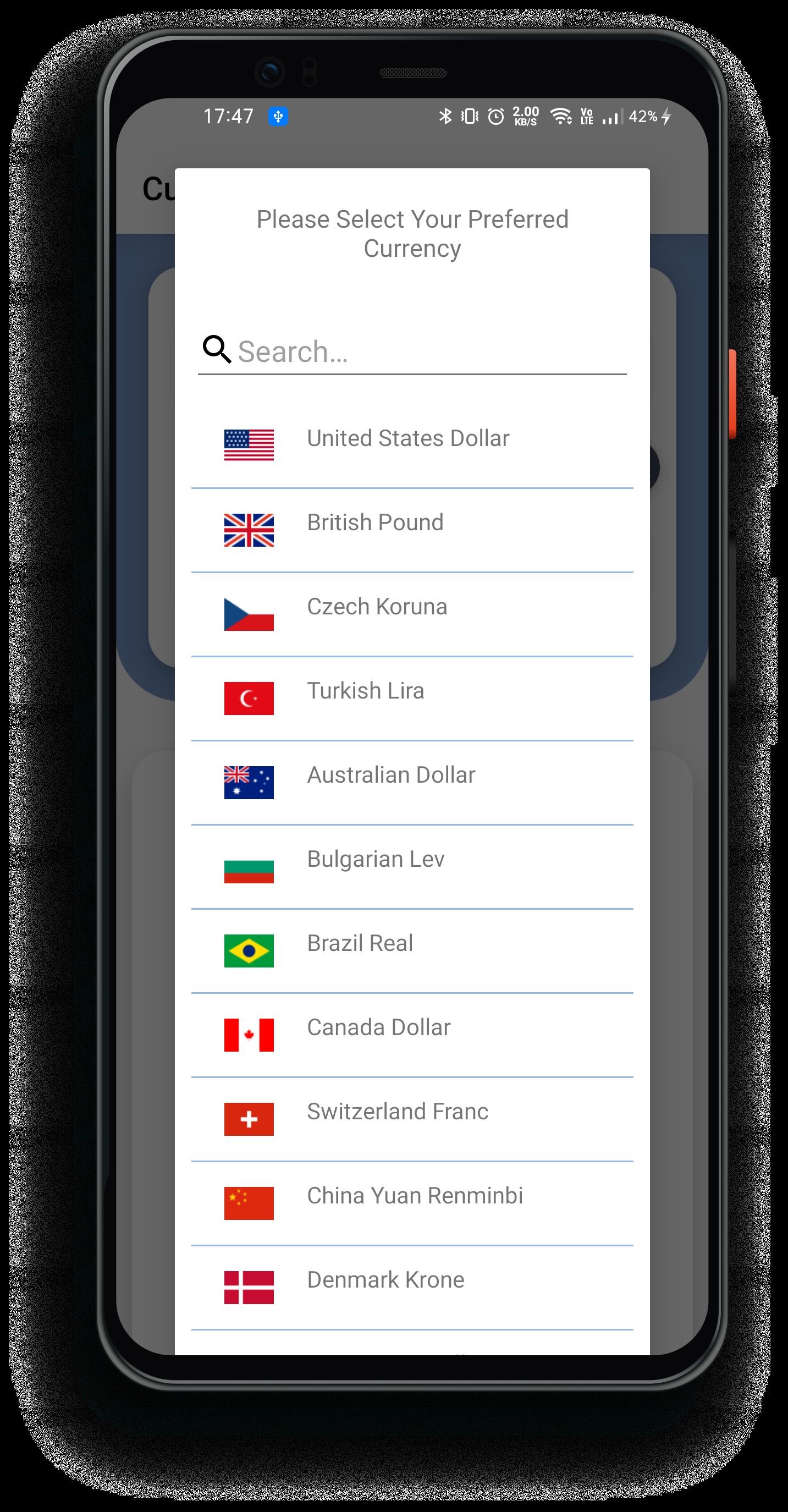A close-up image of a smartphone screen shows the user in the process of selecting their preferred currency for an application, possibly for a financial transaction. The phone, encased in a black cover, displays the time as 17:47. The status bar also indicates active Bluetooth and Wi-Fi connections, an alarm clock icon, and a battery level at 42%. 

On the screen, a search bar with a magnifying glass icon and the word "Search" in light blue text on a white background is visible. Below the search bar, a list of currencies is presented, each accompanied by the flag of the respective country on the left side, vividly colored to represent each nation. The currencies listed include:

- United States Dollar (USD) with the American flag
- British Pound (GBP) with the British flag
- Czech Koruna (CZK) with the Czech flag
- Turkish Lira (TRY) with the Turkish flag
- Australian Dollar (AUD) with the Australian flag
- Bulgarian Lev (BGN) with the Bulgarian flag
- Brazilian Real (BRL) with the Brazilian flag
- Canadian Dollar (CAD) with the Canadian flag
- Swiss Franc (CHF) with the Swiss flag
- Chinese Yuan Renminbi (CNY) with the Chinese flag
- Danish Krone (DKK) with the Danish flag

The overall scene is one of a user navigating through their phone, likely selecting a currency for an international financial transaction.